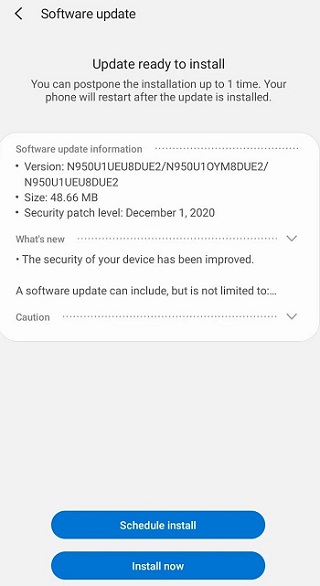Screenshot of a phone device displaying a software update notification. The update, sized at 48.66 MB, features a security patch level dated December 1st, 2020. The main highlight of this update is an improvement to the device's security. The full details are truncated with an ellipsis, suggesting additional information not visible in the screenshot. The screen displays two downward-facing arrows next to labels "What's New" and "Caution," indicating expandable sections. There are two prominent blue buttons: one labeled "Schedule Install," allowing the user to postpone the update once, and another labeled "Install Now," for immediate installation. A notification mentions the phone will restart after the update is installed. The user is likely considering postponing the installation, evidenced by the option to delay the update.